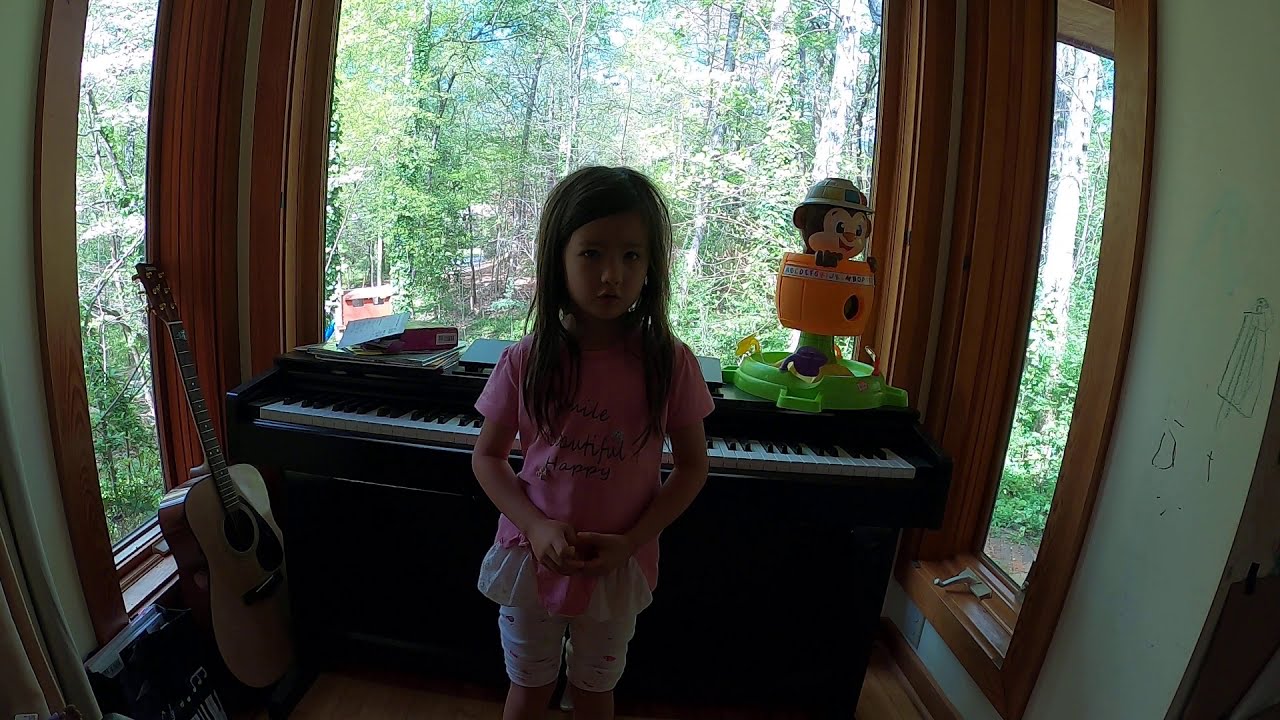The image is a horizontally aligned rectangular photograph of a young girl standing in front of a piano. The girl, who has long, straight dark brown hair pulled over her shoulder, is wearing a light pink shirt with a white and pink ruffled hem and black printed words including "beautiful" and "happy." She is also wearing white shorts that come just above her knees. The girl is looking directly at the camera with her mouth slightly open and her hands together in front of her.

Behind the girl is a black and white piano keyboard. To the left of the keyboard, a brown guitar is leaning against a window. On top of the piano, there is a toy with a green base and an orange barrel-shaped body, resembling a character with a hat.

The background includes a large window with a brown frame behind the girl, and another window on the left side. These windows let in ample natural light, illuminating trees with green leaves outside. Additionally, the wall to the right of the image appears to be an older white wall with drawings made with pen or crayon. The floor is a brown hardwood texture. 

The bright natural light outside contrasts with the indoor scene, highlighting the detail within the room and casting the background into high relief.